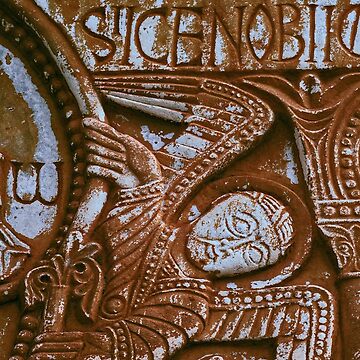The square image depicts a detailed section of what appears to be an ancient carved artwork, resembling a piece one might find on the facade of an old European church. The material, possibly originally a grayish stone like marble, now exhibits significant rust and oxidation, giving it a weathered brown appearance. At the top of the image, engraved into a horizontal metal rectangle, are the partially obscured letters "S-I-C-E-N-O-B-I-I." Beneath this inscription, the artwork features a finely carved angel with bird-like wings. The angel, positioned horizontally in the composition, displays a serene expression with wide eyes. It grasps a circular object with its right hand and holds a staff-like item in its left. To the right of the angel, there's a smaller carving of a bird with its wings spread. The entire piece is interspersed with areas covered by a white, light-blue substance, contributing to its corroded, timeworn aesthetic.